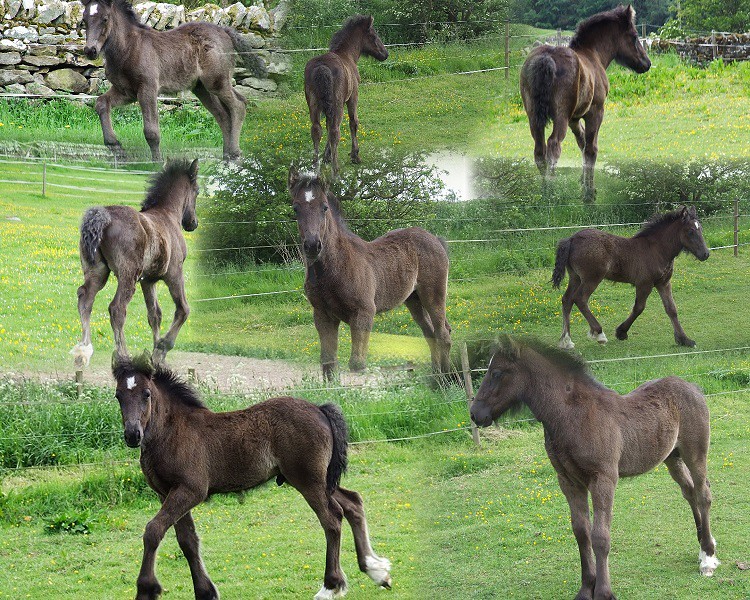The image is a detailed color photo collage consisting of nine faded, interconnected photographs of a dark brown colt with a spiky black mane and tail, adorned with a distinctive white star on its forehead and white fur around its rear hooves. The collage is arranged in three rows with three images per row. The young horse is depicted performing various activities within a grassy, fenced meadow that features a gray stone wall and bushes in the background. Each vignette captures the colt from different angles: standing still, walking, and in mid-run. There is a wire fence visible in multiple images, contributing to a sense of continuity across the scenes. The front hooves of the colt remain dark, and its black nose is a notable feature.